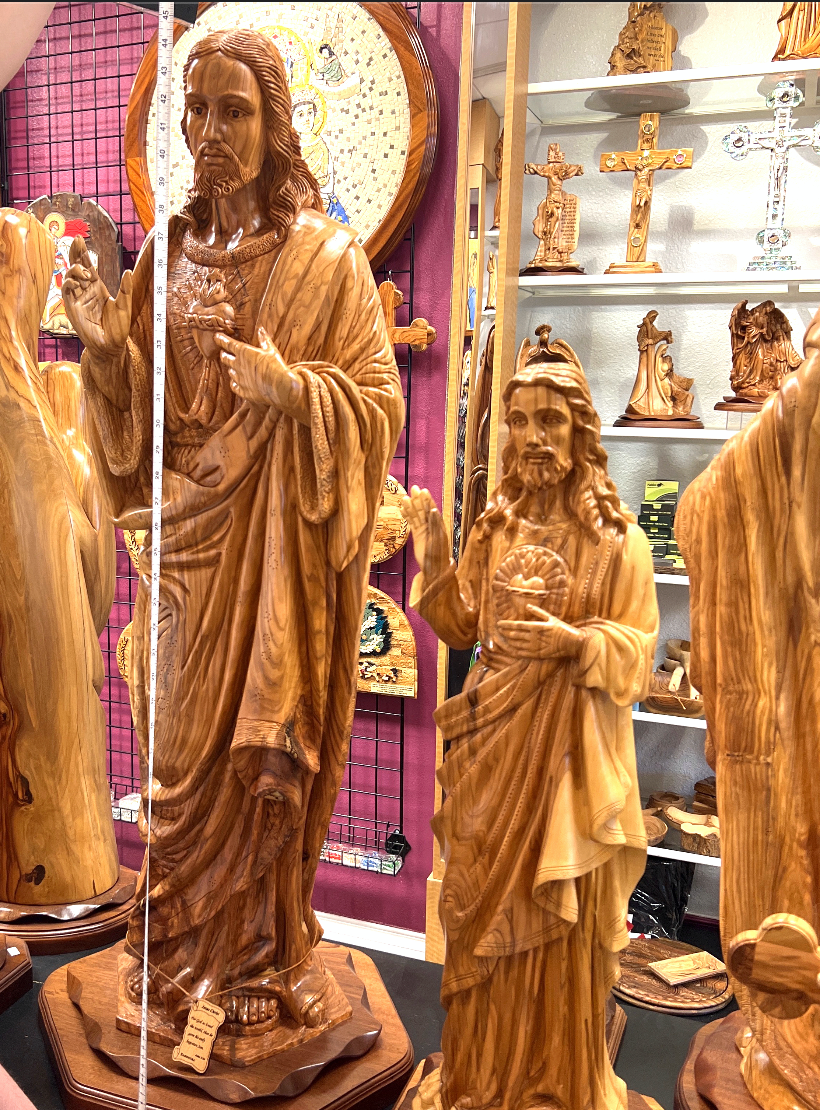The photo features an array of intricately carved wooden statues of Jesus Christ displayed in a retail store. Dominating the scene is a large wooden statue standing approximately 45 inches tall, with a tape measure held up to verify its height. Jesus is depicted with long hair, wearing sandals and a robe, his left hand centered over his chest and his right hand raised in a gesture of greeting. To the left, a seven-foot-tall statue mirrors this pose, while smaller statues are positioned around it. None of the statues are painted; they retain their natural wooden finish, possibly stained. The background showcases a burgundy wall adorned with various other religious images and a rack holding wooden crosses and smaller sculptures. White plastic shelving on the right displays additional religious figurines and scenes, further emphasizing the shop-like environment. The detailed craftsmanship of the statues includes carved representations of the heart of Jesus, underscoring the skill and artistry involved in their creation.